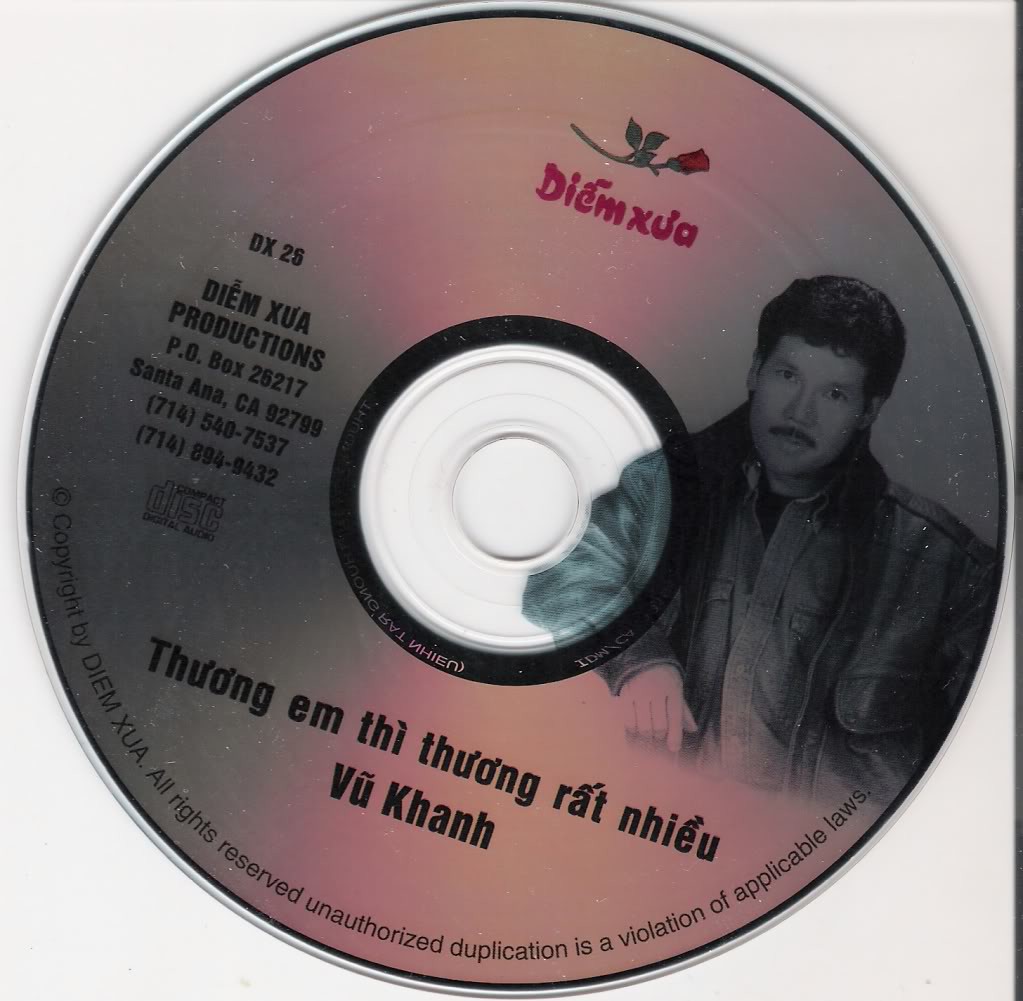This image features a CD with a distinctive color pattern, fading from pink at the top and bottom to gray on the sides. On the right side of the disc, there is a black and white picture of a young man with short black hair and a dark mustache, wearing a jacket. At the top of the CD, there is an image of a rose. The text on the disc includes "DMZua Productions, PO Box 26217, Santa Ana, CA 92799," along with phone numbers "714-540-7537" and "714-894-9432." The text also displays "DMZua" or "Diem Xua" prominently, and indicates it is a Compact Disc Digital Audio. Additional text, some in another language, appears under the central hole of the CD. The bottom of the disc features a copyright notice: "Copyright by DMZua. All rights reserved. Unauthorized duplication is a violation of applicable laws."